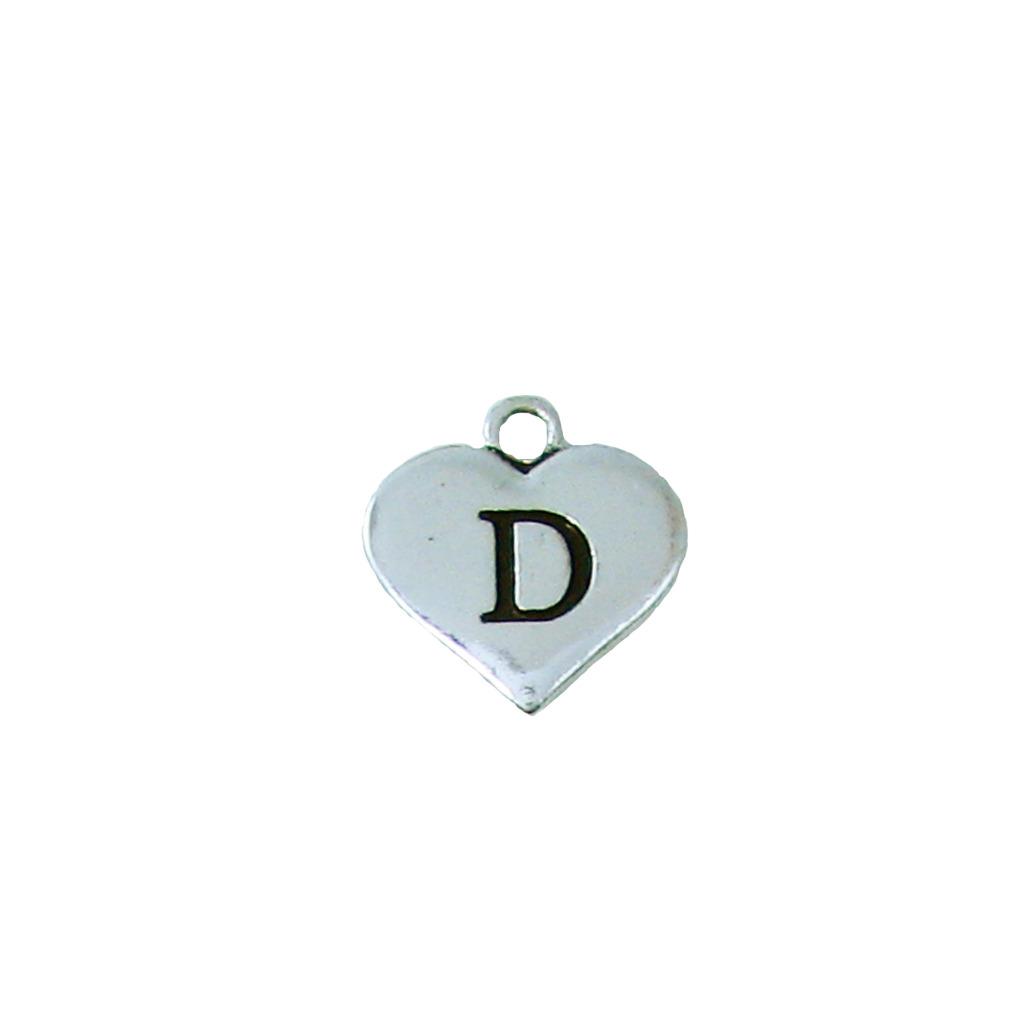The image depicts a small, metallic pendant in the shape of a shiny, reflective silver heart against a pure white background. The heart features a large, capital letter "D" engraved in black at its center. At the top of the pendant, there is a small hole or latch designed for attaching it to a necklace chain. The simple composition focuses solely on the intricately detailed heart-shaped pendant and its engraved letter, highlighting its reflective silver surface and the black letter D.